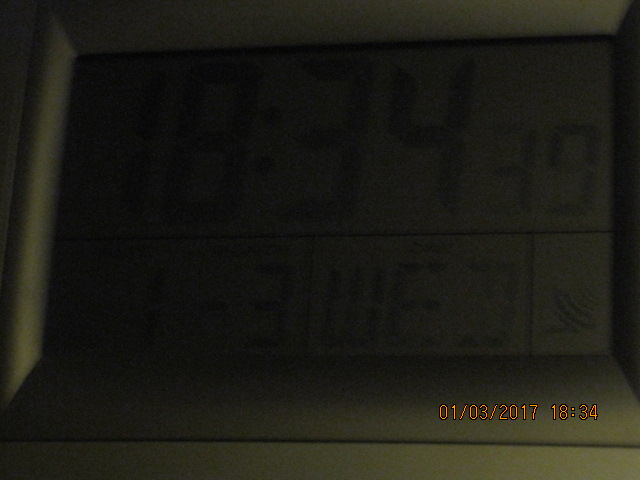In this close-up photograph, the focal point is an old digital clock encased in a dark gray plastic border, which frames an equally dark gray screen. The digital clock displays the time as "18:34" with somewhat unclear seconds that appear to be either "30" or "39" due to the blurriness of the image. Below the main time display, there is a thin horizontal line, beneath which a long rectangular section on the left side reads "-3". Adjacent to this, another box contains the letters "WE," and a third box on the right side appears empty. In the bottom right-hand corner, dated "01-03-2017" in sketchy yellow text with a black border, the time "18:34" is repeated next to it. The entire image is notably blurred, making it challenging to discern finer details clearly.